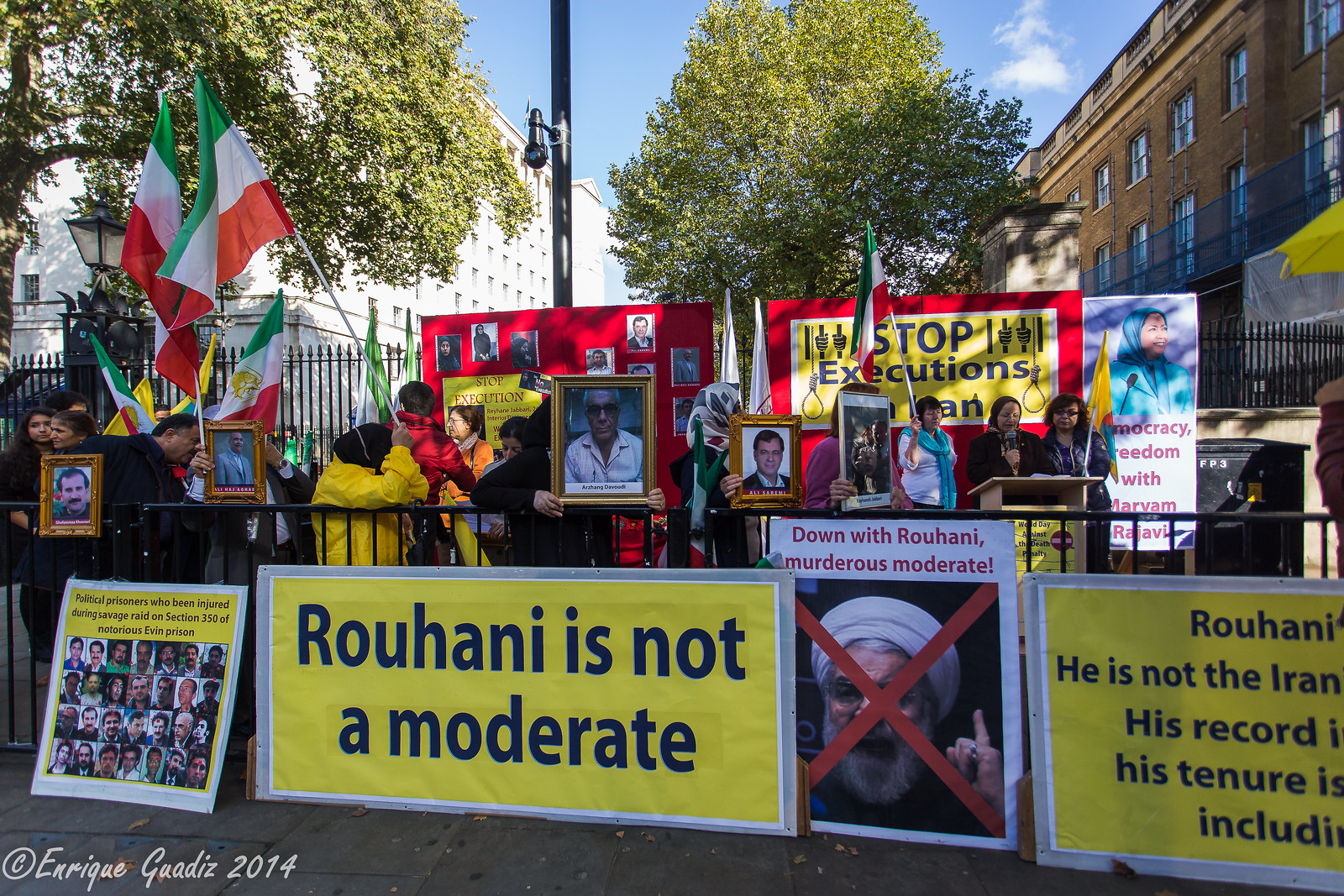In this vibrant city scene, a significant demonstration is taking place under a clear blue sky with large trees and tall buildings flanking the scene. At the forefront, there is a prominent yellow sign with a white border that asserts, "Rouhani is not a moderate." Several people are carrying large framed photographs, some of which are marked with a bold red X, suggesting they are victims allegedly associated with Rouhani. The demonstrators hold flags characterized by three horizontal stripes of green, white, and red, possibly representing their national identity. Interspersed among the crowd are additional signs with various backgrounds and messages, including a noticeable yellow sign that demands, "Stop executions." A metal fence can also be seen behind the demonstrators. This visual amalgamation of posters, signs, and flags underscores the collective outcry against what appears to be oppressive actions attributed to Rouhani, making it a poignant scene of protest and remembrance.